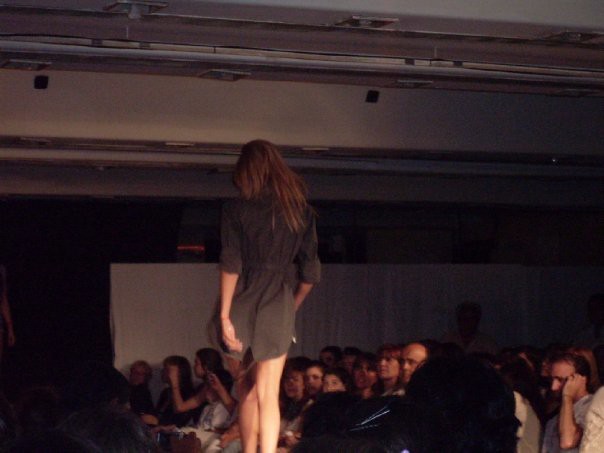In this image, a woman is the main focus, confidently striding down a dimly lit catwalk, giving prominence to her modeling a short, black dress that accentuates her shapely legs, almost up to the buttocks. Her long, light brown hair cascades down her back as she poses, possibly indicating a beauty pageant or a fashion show setting. The event appears to be in a low-ceilinged, basement-like room with a basic ceiling and exposed pipes. The audience, comprised of several individuals including a distinct bald man with glasses and a young girl around 11 or 12 years old with her left hand raised, looks on with mixed expressions. The scene is illuminated mostly by stage lights, casting a dramatic focus on the model while keeping the rest of the room relatively dim. Subdued colors like white, gray, brunette, black, and hints of other neutral tones dominate the scene. The ambiance suggests either a casual or somewhat underground fashion display with a hint of intrigue and mystery.